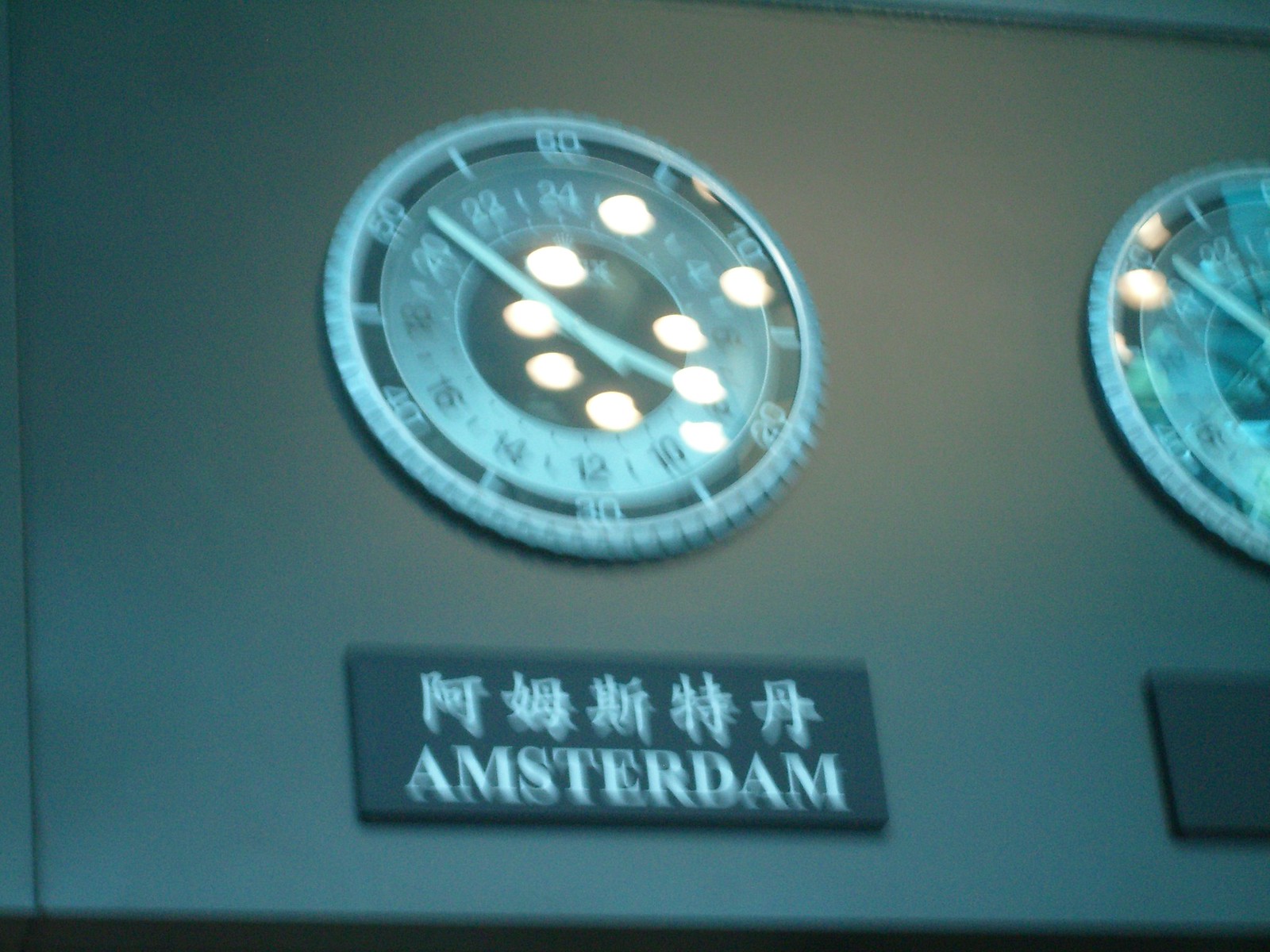The image depicts a blurred clock designed to display times from different countries or time zones. The specific clock in focus appears to show the current time for Amsterdam, accented by Asian characters, which may suggest an additional cultural or functional context. The clock face features nine circular lights, possibly for extra illumination or indicators. It has two visible hands, similar to a standard clock, but the presence of a second hand cannot be confirmed due to the blurriness. Notably, it operates on a 24-hour cycle, starting at 1 and ending at 24.